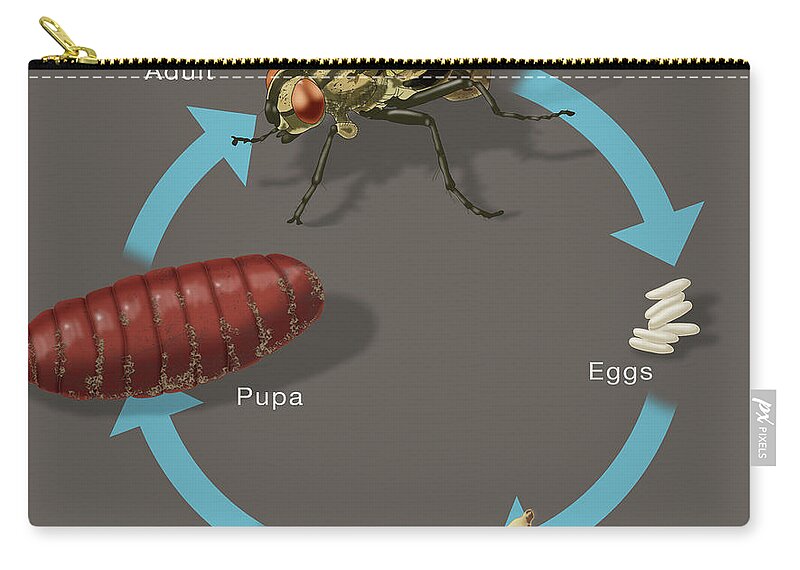The image in question appears on a gray, rectangular zip-up pouch, perhaps used for money, cosmetics, or pencils. The image, styled in a painterly and scientific manner, illustrates the life cycle of a common housefly in a triangular pattern with circular blue arrows connecting each stage. The sequence starts with white, oval-shaped eggs on the right side, transitions downwards to the reddish-brown, cigar-shaped pupa in the center, and then moves to the top left where the adult housefly is depicted. The housefly has a greenish body with red, copper-colored eyes and black legs. The clear, educational diagram stands out against the muted gray background of the pouch, with the golden-colored zipper adding a contrasting decorative touch.